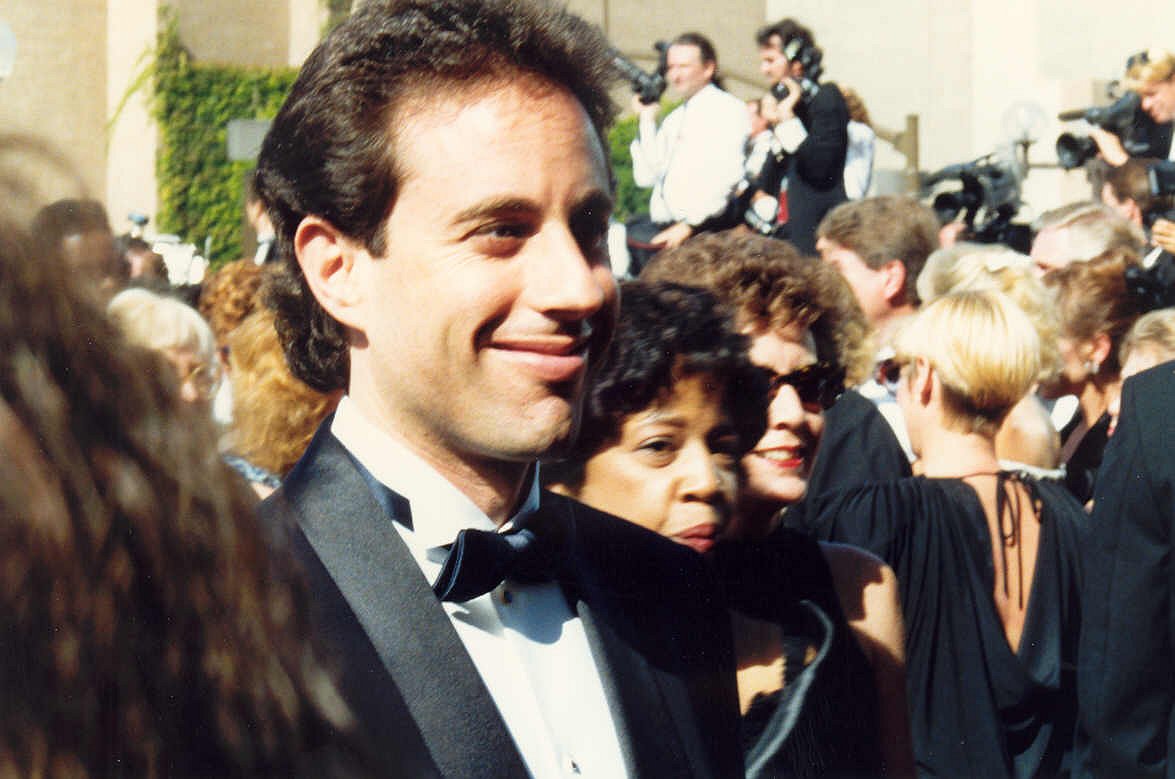This vintage daytime photograph captures a smiling Jerry Seinfeld on a red carpet at a formal event. Jerry, a white male with dark hair and a receding hairline, is elegantly dressed in a black tuxedo, white shirt, and black bow tie. He stands out in the center of the image, looking to his right. The scene is bustling with formally dressed men and women of varied hair colors, primarily in black attire. Closest to him on the left, partly out of focus, is a person with dark brown hair. On his right, there is a black woman with short dark hair and a Caucasian woman with lighter brown hair wearing sunglasses. Behind them, more people can be seen, including two photographers in the distant background. The backdrop features a large white building adorned with green vines. The sunlight touching the crowd and surroundings further enhances the warm, nostalgic feel of the photograph.